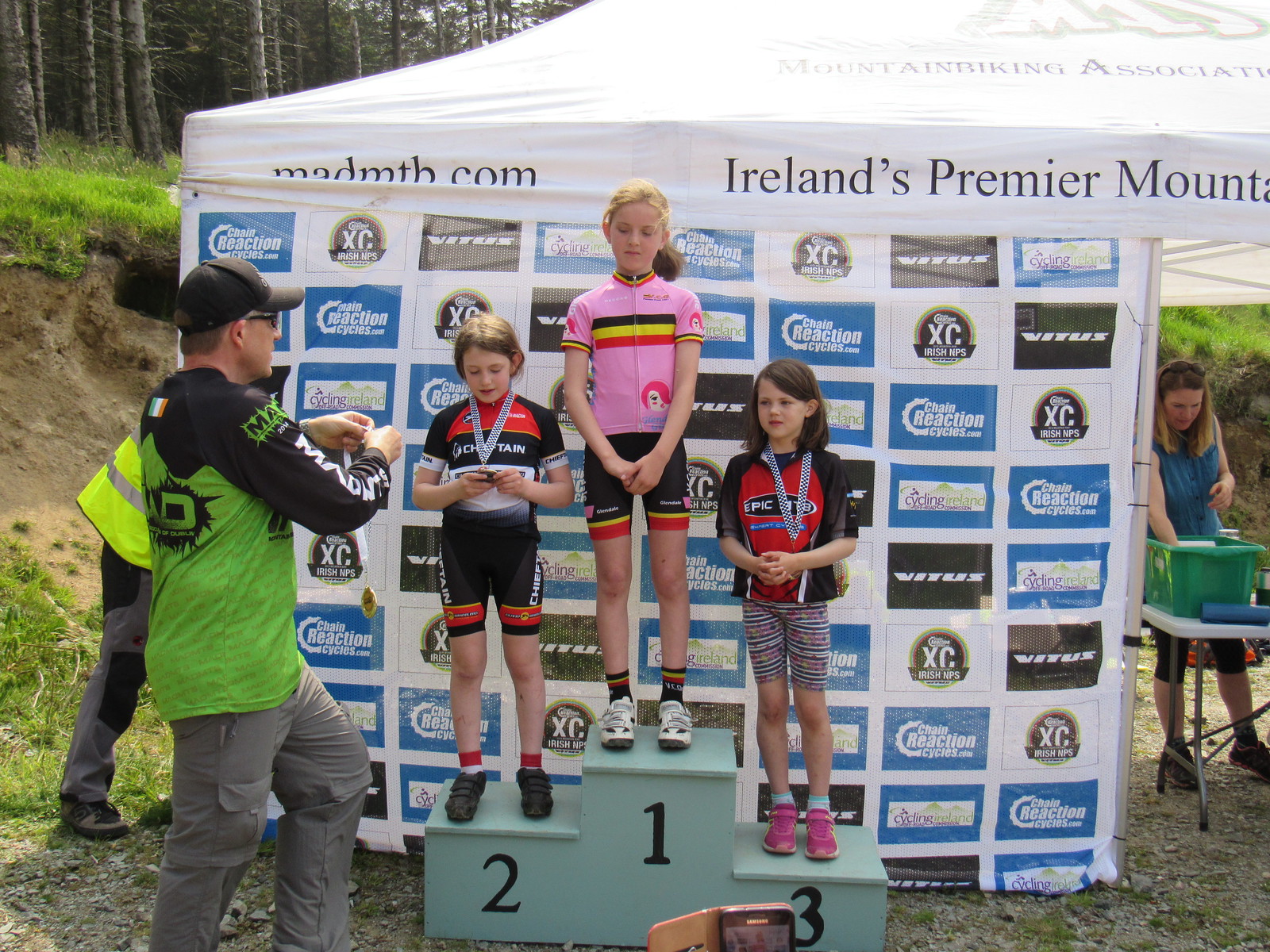In this image, three young children, likely under the age of nine or ten, stand proudly on a green winner's podium after completing a race or athletic event. The girl in the middle, positioned on the "1" podium, wears a pink shirt with black, yellow, and orange stripes and black shorts, and she has blonde hair. She looks down as a man, dressed in a yellow-green shirt and gray pants, approaches to award her a medal. To her left on the "2" podium, a girl with brown hair wearing a black and red shirt and shorts examines her already awarded medal, while on the "3" podium to the right, another girl in a red and black shirt and pink shoes stands with her medal around her neck.

The event takes place outdoors against a backdrop featuring a white tent adorned with numerous advertisements and a prominent sign that reads "Ireland's Premier Mountain..." though the rest of the text is obscured. In the vicinity of the tent to the right, a lady sorts through a green bin behind a table, suggesting a volunteer area. The setting is adjacent to a wooded area with a slight hillside visible in the background.